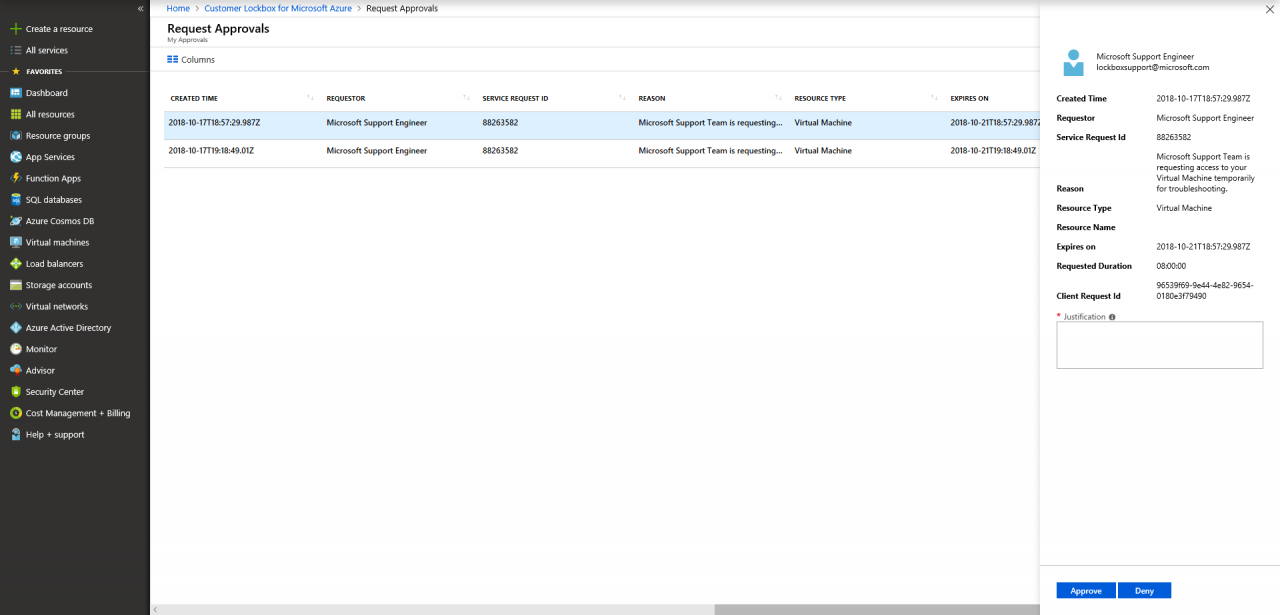A detailed page from a Microsoft Azure web application is displayed. At the top, the navigation bar includes options such as "Home," "Customer Lockbox for Microsoft Azure," and "Request Approvals." The main body of the page focuses on "Request Approvals," listing two items with detailed information. Each item includes the "Created Time" marked as "2018-10" followed by a series of numbers, the designation of "Microsoft Support Engineers" as the requester, a "Server Request ID," the reason for the request by the Microsoft Support Team, the type of resource involved (a virtual machine), and the expiration date of the request.

On the left side of the screen, there is a vertical black column presenting various selectable options including "Create a Resource," "All Services," "Your Favorites," "Your Dashboard," "Resource Group," "App Services," "Function Apps," "Virtual Machines," and "Load Balancers."

To the right of the main content, a white box is open displaying specific details about the request from the Microsoft Support Engineer. This section contains the name of the engineer, the creation time of the request, the requester details, the service request ID, and the reason given for the access request, which is to temporarily access the user's virtual machine for troubleshooting purposes. Additionally, there is a "Client Request ID" listed in this section.